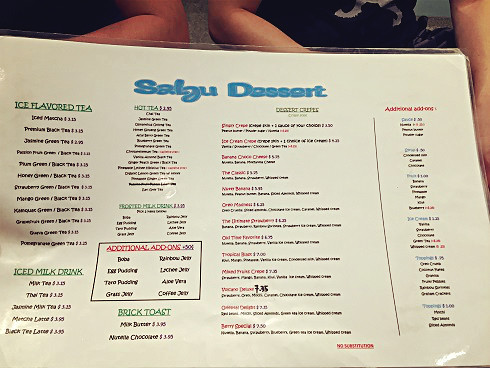The image displays a large, laminated diner menu titled "Sell You Dessert," with the header written in bold blue text. The menu features a variety of dessert items, although the specific names and details are difficult to discern due to the blurred red and black text. Among the desserts, faint images of ice cream cones are visible. On the left side of the menu, an array of flavored iced teas is listed, including options like iced mocha, honey, and mango. Below the flavored iced teas, the menu presents different iced milk teas featuring varieties such as Thai tea and black tea, along with their respective prices. The overall presentation suggests a dessert-focused selection with a diverse range of iced beverages.